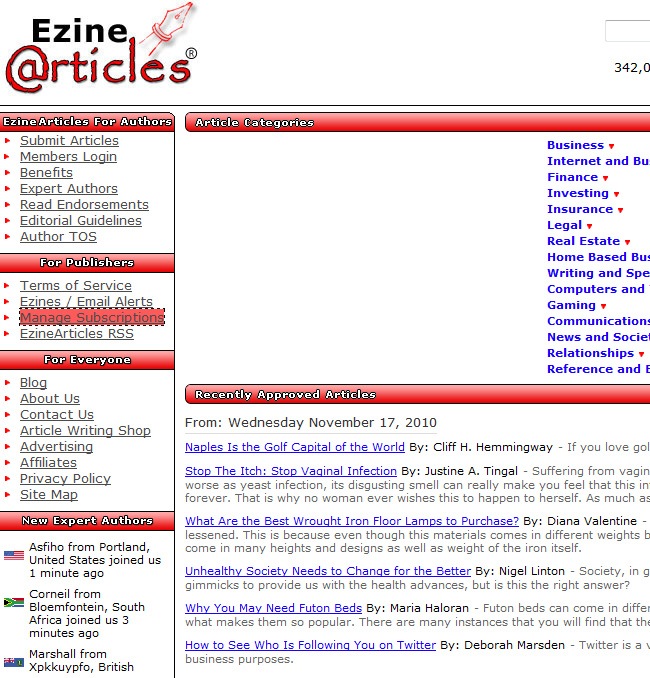A screenshot of the website "Ezyne Articles" is depicted. In the top left corner, there is the site name with "Ezyne" in black and "Articles" in red. The 'A' in "Articles" is stylized to resemble an @ symbol, encircled by a line. Right next to this, there's a small red doodle of a pen.

Below this, a left-hand navigation pane displays several headers and their respective links. The first header, "Ezyne Articles for Authors," includes the links: "Submit Articles," "Members Login," "Benefits," "Expert Authors," "Read Endorsements," "Editorial Guidelines," and "Author TOS." The next header, "For Publishers," has the links "Terms of Service," "Ezyne Email Alerts," "Managed Subscriptions," and "Ezyne Articles RSS." Under "For Everybody," the links listed are "Blog," "About Us," "Contact Us," "Article Writing Shop," "Advertising," "Affiliates," "Private Policy," and "Sitemap." The final header, "New Expert Authors," showcases three flags below, indicating new users.

The "Managed Subscriptions" section is currently selected, revealing a large section to its right titled "Article Categories" featuring hyperlinks including "Business," "Finance," "Investing," "Insurance," "Legal," "Real Estate," and "Gaming", with additional categories partially cut off from the page view.

Further down the page, under the heading "Recently Approved Articles," several article titles are listed with their publishing date, Wednesday, November 17th, 2010. These titles include:
- "Naples is the golf capital of the world"
- "Stop the itch, stop vaginal infection"
- "What are the best route iron floor maps to purchase"
- "Unhealthy societies to change for the better"
- "Why you may need futon beds"
- "How to see who is following you on Twitter"